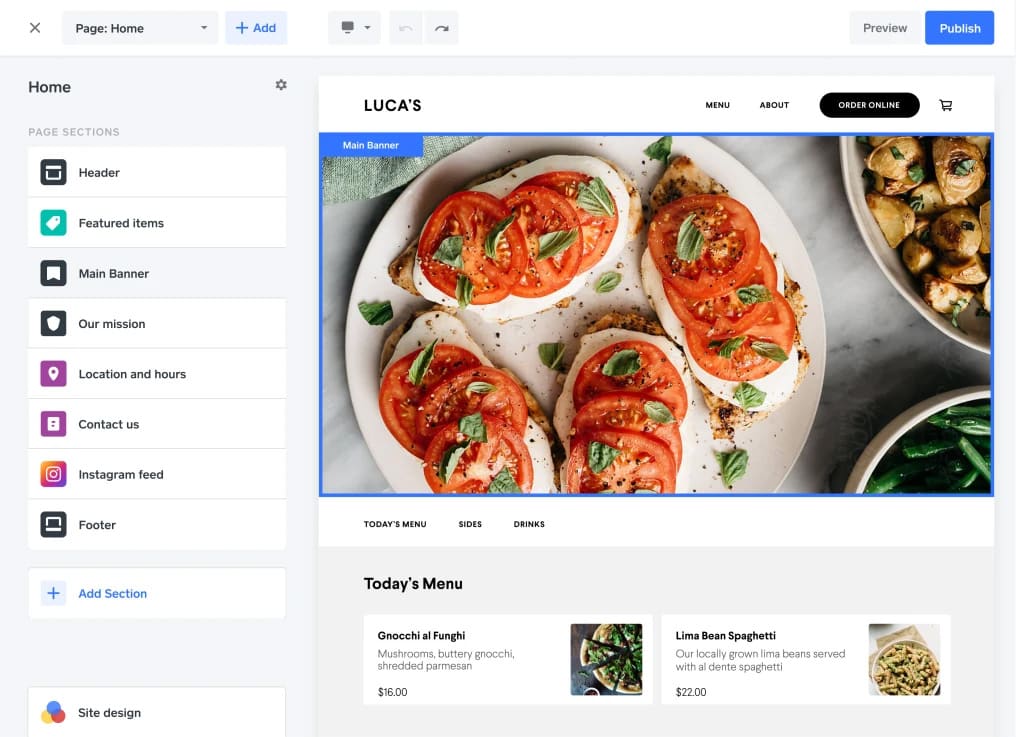The image is a screenshot of a webpage, specifically a menu page. At the top left of the screen, there is navigation text that reads "Page Home" followed by "Plus Add." Adjacent to this, there's an icon of a monitor with a down arrow button next to it, along with back and forward buttons.

In the upper-right corner, there are two buttons: "Preview" and "Publish," with the "Publish" button highlighted in blue.

Down the left-hand side, there's a vertical menu starting with "Home" featuring a settings gear symbol next to it. Below this, there are several sections listed: "Page Sections," "Header," "Featured Items," "Main Banner," "Our Mission," "Location and Hours," "Contact Us," "Instagram Feed," and "Footer." Below these sections, there's a blue button with a plus sign labeled "Add Section."

At the bottom of this left sidebar, there are three interconnected circles in blue, red, and yellow with the label "Site Design."

On the right side of the screen, there's a large image of a dish that appears to be a Caprese toast or a similar creation, featuring tomato slices and basil atop provolone cheese. The dish is served on either toast or chicken breast, presented on a white plate. In the top corner of the plate, there are rosemary potatoes, and at the bottom right corner, some green beans are visible.

Below this image, there is text that reads "Luca's" and navigation options such as "Menu," "About," and "Order Online." Further down, there is a section titled "Today's Menu" featuring options like "Gnocchi alla Funghi" and "Lima Bean Spaghetti."